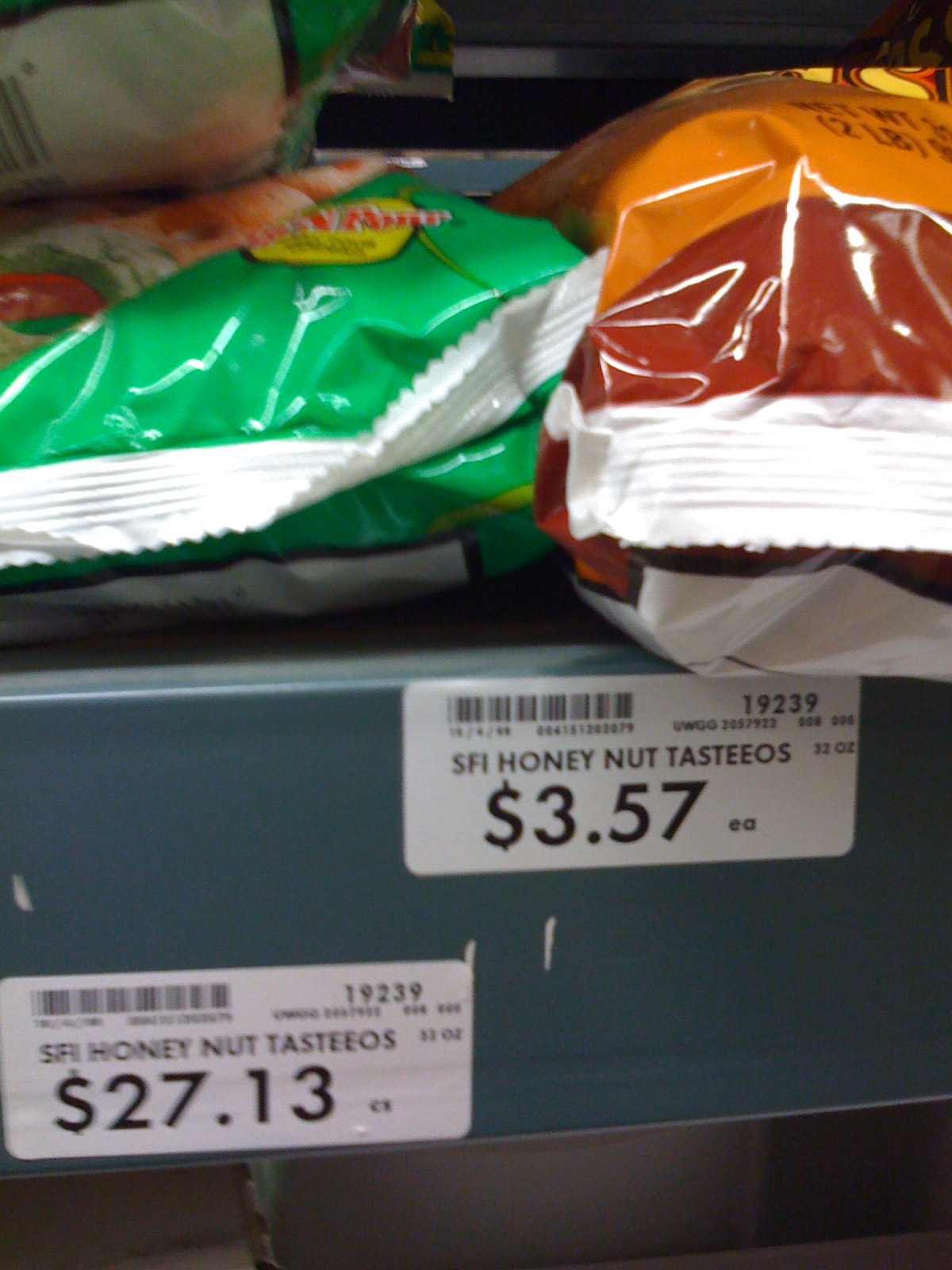This close-up photograph captures two vacuum-sealed product bags lying on their backs on a store shelf, seemingly squished together at the center of the image. The bag on the left, positioned towards the top of the image, is dark green with hints of yellow, black, and possibly a real-life image of the food item inside, though the details are obscured by the crumpled packaging. This green bag also features a white tab where it is sealed.

To the right, another bag shares the same position and is orange with maroon accents. It also has a white tab at the sealing point. Partial yellow text on this bag reveals "2 LB net weight," visible at an angle.

Beneath these bags, the dark blue store shelf displays two white rectangular price tags with black text. The tag under the green bag reads "SFI Honey Nut Tasty O's" followed by a barcode, the code number "19239," and the price "$3.57 each." Slightly to its left, another tag also reads "SFI Honey Nut Tasty O's" but lists the price as "$27.13 each." Below the shelf, the image reveals some grey-white textures, although this area is mostly shadowed.